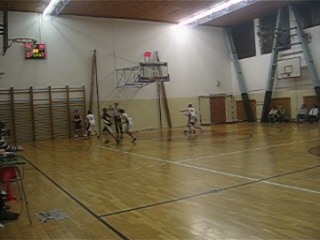The image is a small, rectangular photograph taken inside what appears to be a school gymnasium, viewed in landscape orientation. The gym features three basketball hoops: one on the far left, one on the far right, and another almost perfectly centered. The gym floor is light wood with various lines marking different sports boundaries. In the upper left corner, a scoreboard is attached to the white back wall, though the scores are illegible. The ceiling is a brown hue, but it is brightly lit, illuminating the entire space. Near the far end of the gym, several young people and possibly a referee are gathered, though specific details about their actions or who has possession of the ball are unclear.